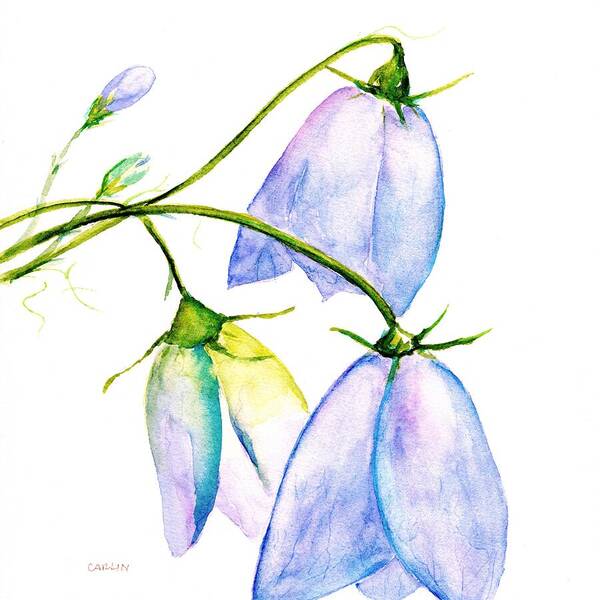This delicate watercolor illustration, signed "Carlin" in the lower left corner, exquisitely depicts several flowers against a plain white background. The main focus comprises three flowers with slender green stems, gracefully drooping like pendant lights. Their petals, a blend of bluish-purple hues with blue shadowing and white reflections, create a translucent appearance that allows light to gently permeate through. Each flower showcases three delicate, oval-shaped petals. Above these blooms, two erect buds, yet to open, add a sense of potential and freshness to the scene, while their delicate translucency hints at the ephemeral nature of these spring wildflowers. The artistry captures the fragile beauty and transient existence of these blossoms, highlighted by their intricate, light-filled petals and subtle hints of yellow in the leaves.